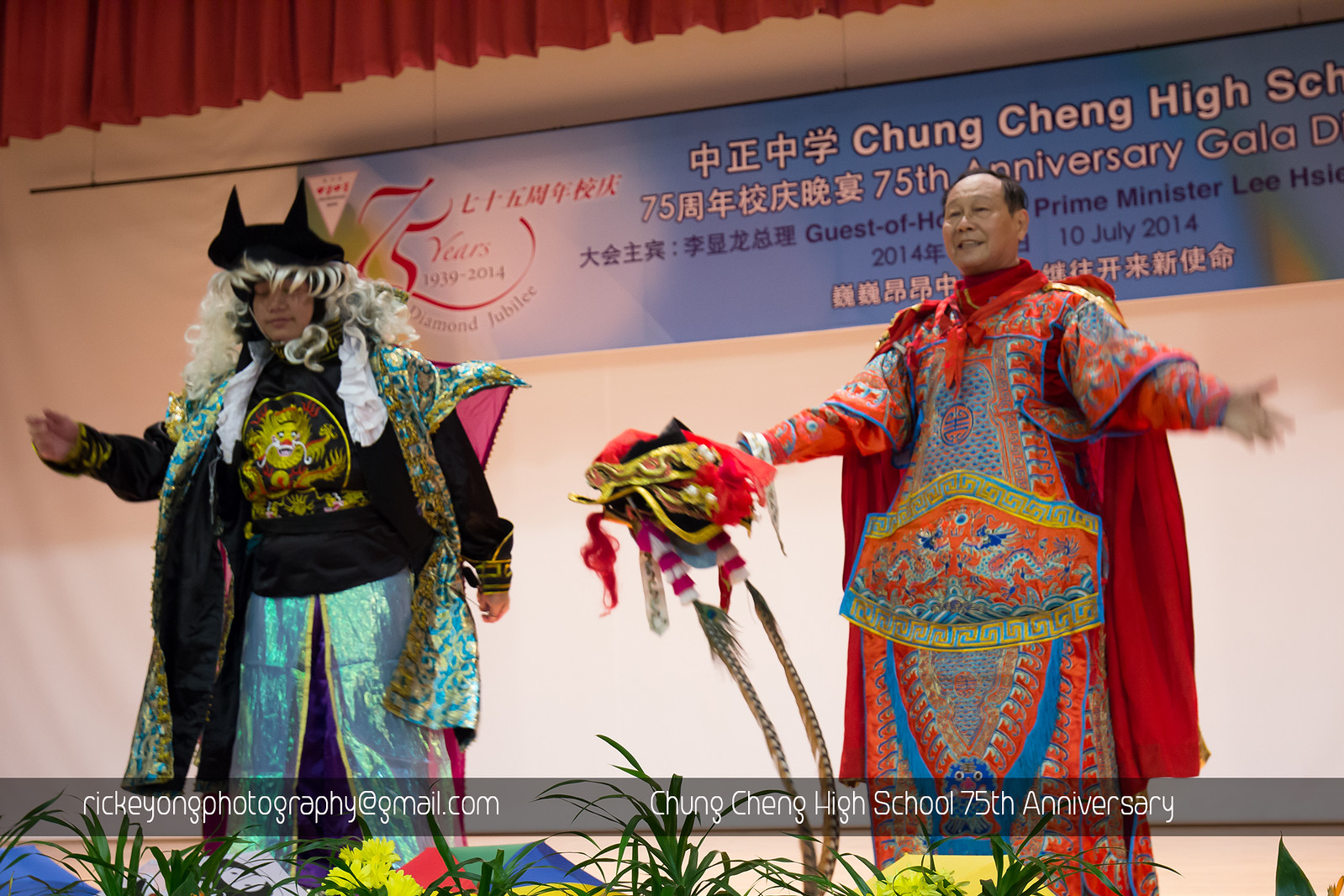The image captures two Asian men on a stage during the Chung Cheng High School 75th Anniversary Gala. They are dressed in vibrant, colorful costumes reminiscent of Japanese garb. 

The man on the left is dressed in an elaborate costume featuring a hood with ears on it, fur on the sides, and a black top adorned with an embroidered gold lion. He also has a multicolored shiny green and blue bottom, giving a striking appearance that resembles a cat outfit. His attire includes elements of cosplay, with long curly blonde hair peeking out.

The man on the right is wearing an eye-catching red and blue, abstract-patterned outfit. He holds a dragon mask in one hand and has his arms outstretched. Both men are slightly bowing, indicating they might be receiving a presentation or performing. They stand in front of a white wall with a red curtain above and a blue banner in Asian writing. The scene is adorned with flowers at the bottom and includes a watermark that reads "Nick Yang Photography." 

Prominently displayed are signs and banners that mark the significance of the event, stating “Chung Cheng High School 75th Anniversary.”